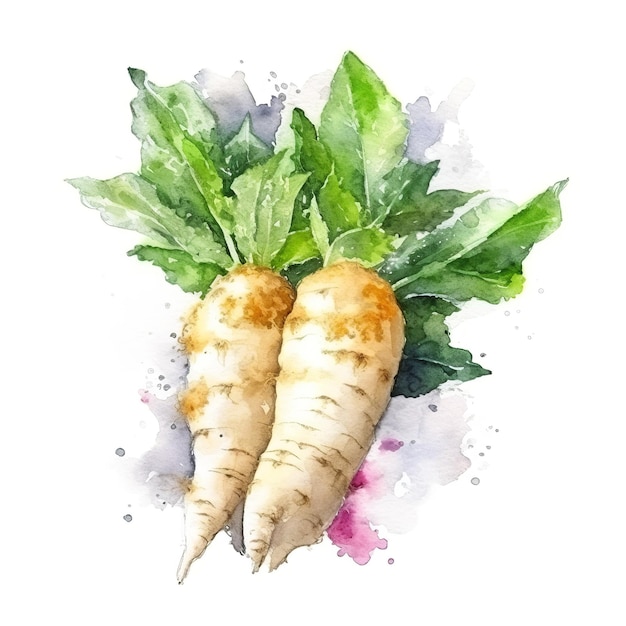This image showcases a detailed watercolor painting of two turnip-like vegetables, possibly radishes or daikon radishes. The main bodies of the vegetables are an off-white, creamy color with light brown patches of dirt, possessing a chunky and substantial appearance. The tubular vegetables feature multiple pointed ends, particularly prominent in the one in the foreground. At the tops, lush green leaves sprout in a bunch, adding vibrant color to the composition. Surrounding the vegetables, the background is adorned with splashes and splotches of magenta, light purple, and pink watercolor paint, creating a dynamic and textured contrast against the plain white backdrop. Additionally, there are small speckles of paint scattered around, enhancing the lively and artistic feel of the painting.